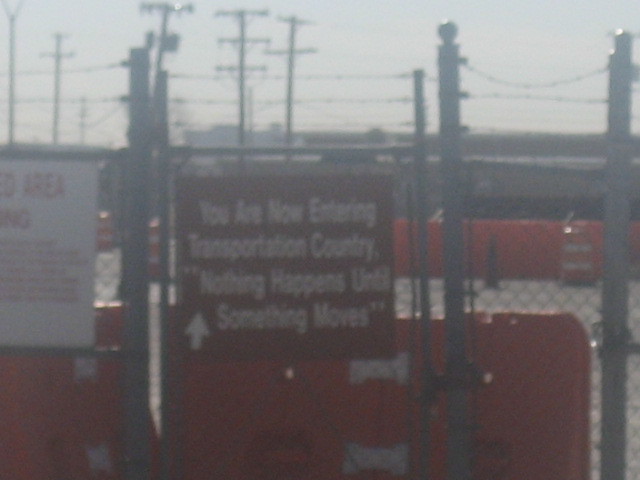A bleak, overcast sky looms above, casting a somber atmosphere over the scene. On the left side of the image, a weathered white sign stands prominently, partially obscured by a robust chain-link fence topped with gleaming silver poles and menacing strands of barbed wire. In the background, a striking red hue dominates the view, with several red traffic cones scattered across the area, visually punctuating the somber gray. 

Amidst this industrial landscape, another sign commands attention, boldly proclaiming, "You are now entering transportation country. Nothing happens until something moves." This statement underscores the significance of movement in this starkly utilitarian environment. The barbed wires, sharply angled upwards, add an element of harshness to the scene.

Further enhancing the industrial vibe, red walls and dividers stretch across the background, interspersed with patches of white, creating a stark contrast. Numerous electrical poles punctuate the setting, their lines converging and diverging, adding to the chaotic yet structured aesthetic of this transportation hub.